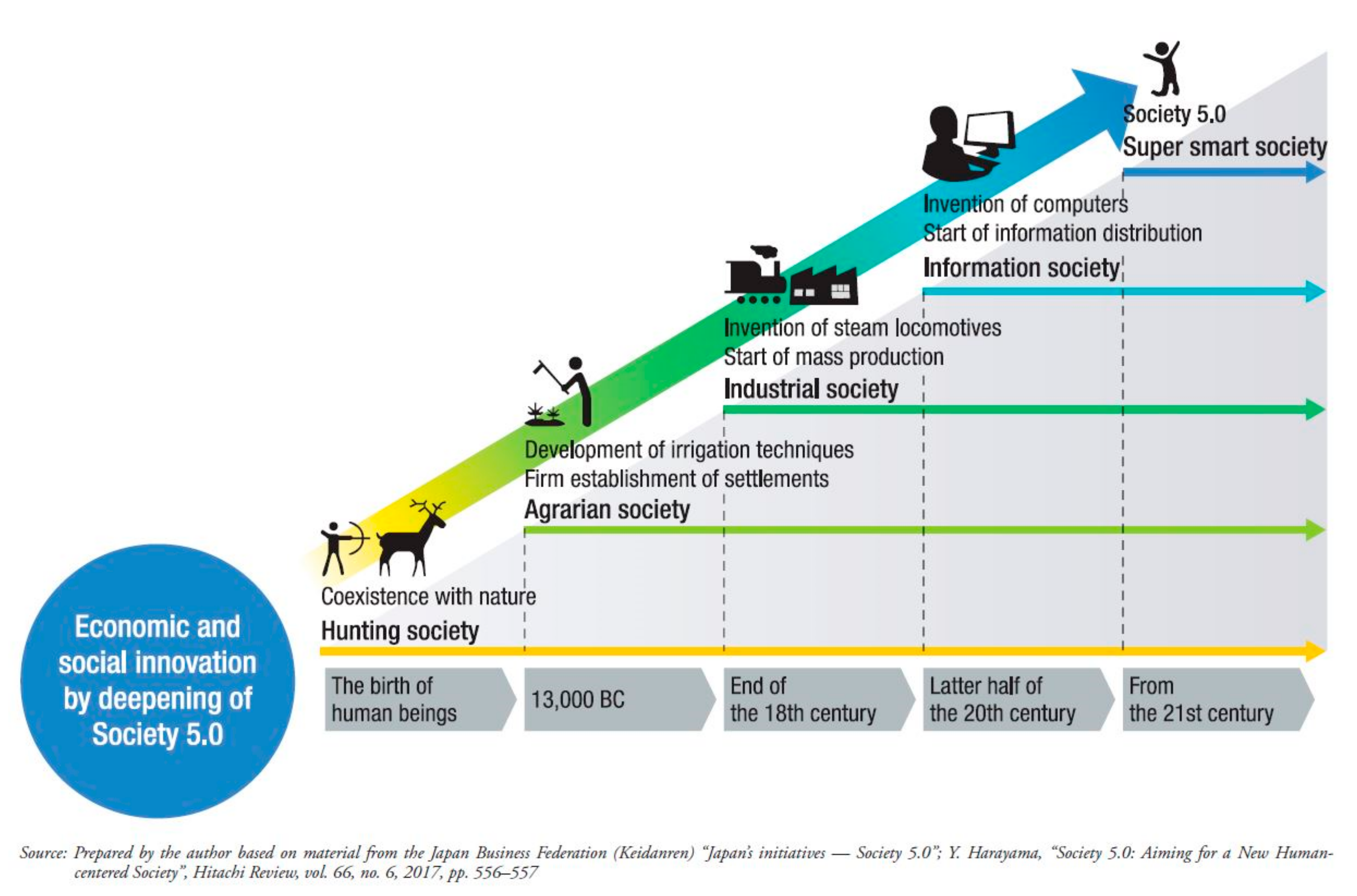The informational image features a computer-generated flowchart on a white background, with a gray chart in the center. The chart displays an upward arrow moving diagonally from the bottom left to the top right, transitioning through a multicolored gradient of yellow, green, teal, and blue. At the top of the chart is the title, "White Tech's Economic and Social Innovation by Deepening of Society 5.0," displayed within a blue circle located in the bottom left corner. The arrow is segmented into five sections, each representing a different historical era and societal advancement. These segments are as follows: 

1. "Coexistence with Nature" dating back to 13,000 BC, highlights the agrarian society and the development of irrigation techniques.
2. "Development of Irrigation Techniques," signifying the end of the 18th century, representing the industrial society with the invention of steam locomotives and the start of mass production.
3. "Invention of Steam Locomotives," leading into the latter half of the 20th century, indicative of the information society marked by the invention of computers and the start of information distribution.
4. "Invention of Computers," progressing from the 21st century onwards, to symbolize Society 5.0, or the super smart society, represented by a small man icon at the top of the chart.

Each section is visually represented by a column that increases in height, illustrating the progression and deepening of societal transformation through different innovations over time.